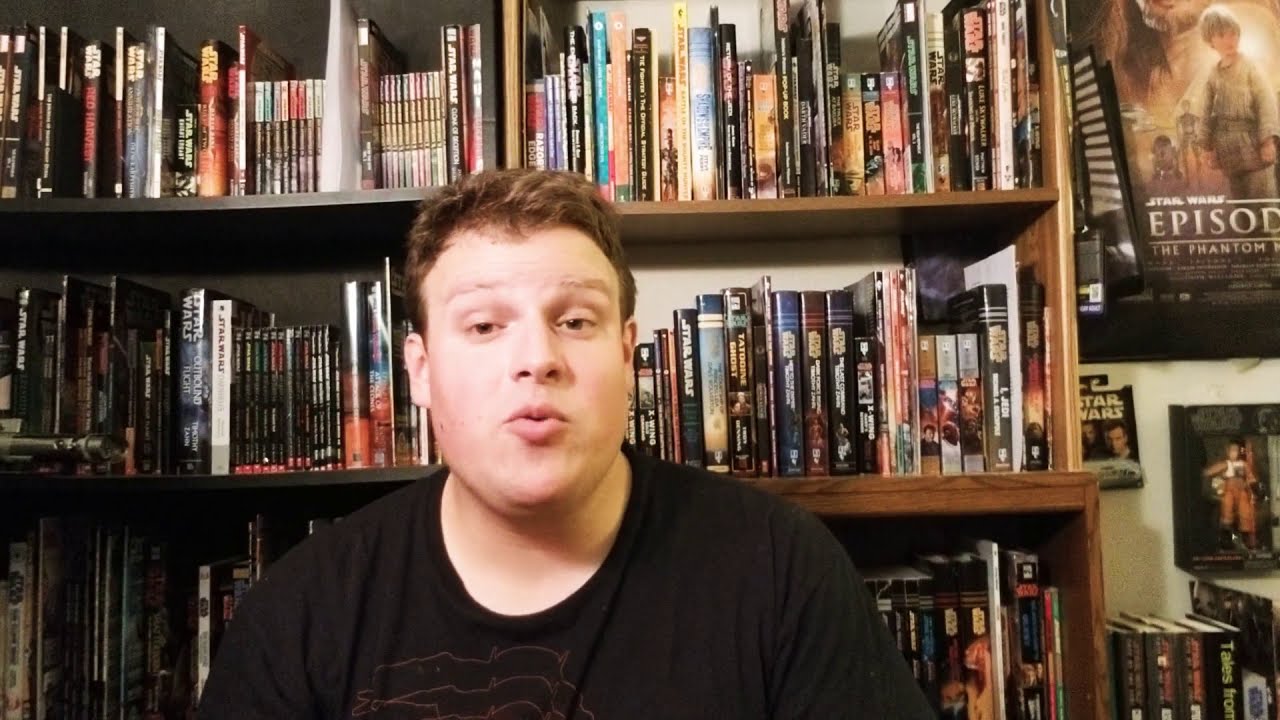The image features a young man who appears to be engaging in a video or podcast, possibly reviewing Star Wars content. He is seated indoors, likely in his house, and faces the camera while mid-sentence. He wears a black short-sleeved shirt with an indiscernible logo. Behind him, a large, well-stocked bookshelf spans three rows, filled with various Star Wars books, CDs, DVDs, and graphic novels, distinguishable by their differing sizes and shapes, with some potentially in different languages. The Star Wars theme extends to the decor, with a prominent Star Wars: The Phantom Menace poster on the wall and additional memorabilia. The room, filled with collectibles, adds to the impression that he's in a personal space dedicated to his interests.